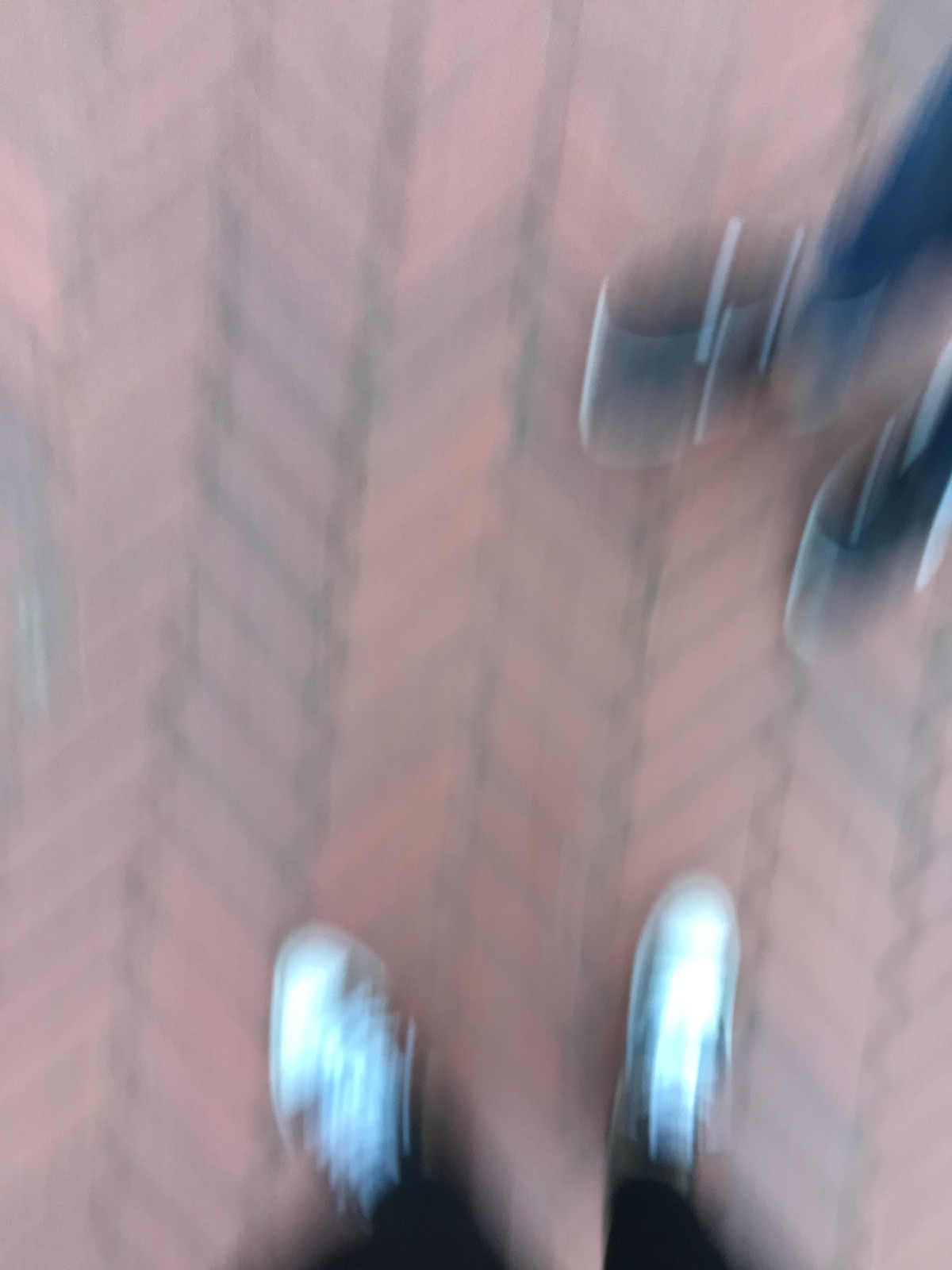In this rectangular image, the photograph is extremely blurry, almost resembling double vision. From our perspective, we are looking downward at the ground. Near the bottom of the image, there are two slightly discernible shoes along with the ankles of a human, seemingly wearing white shoes and dark pants. In the upper-right corner, we catch a glimpse of two more feet and ankles, viewed diagonally. These second shoes appear to be dark in color. Both pairs of feet stand on a brick-paved ground or patio. The red bricks are laid diagonally, creating a chain-link pattern. The image captures approximately six vertical rows of these bricks.